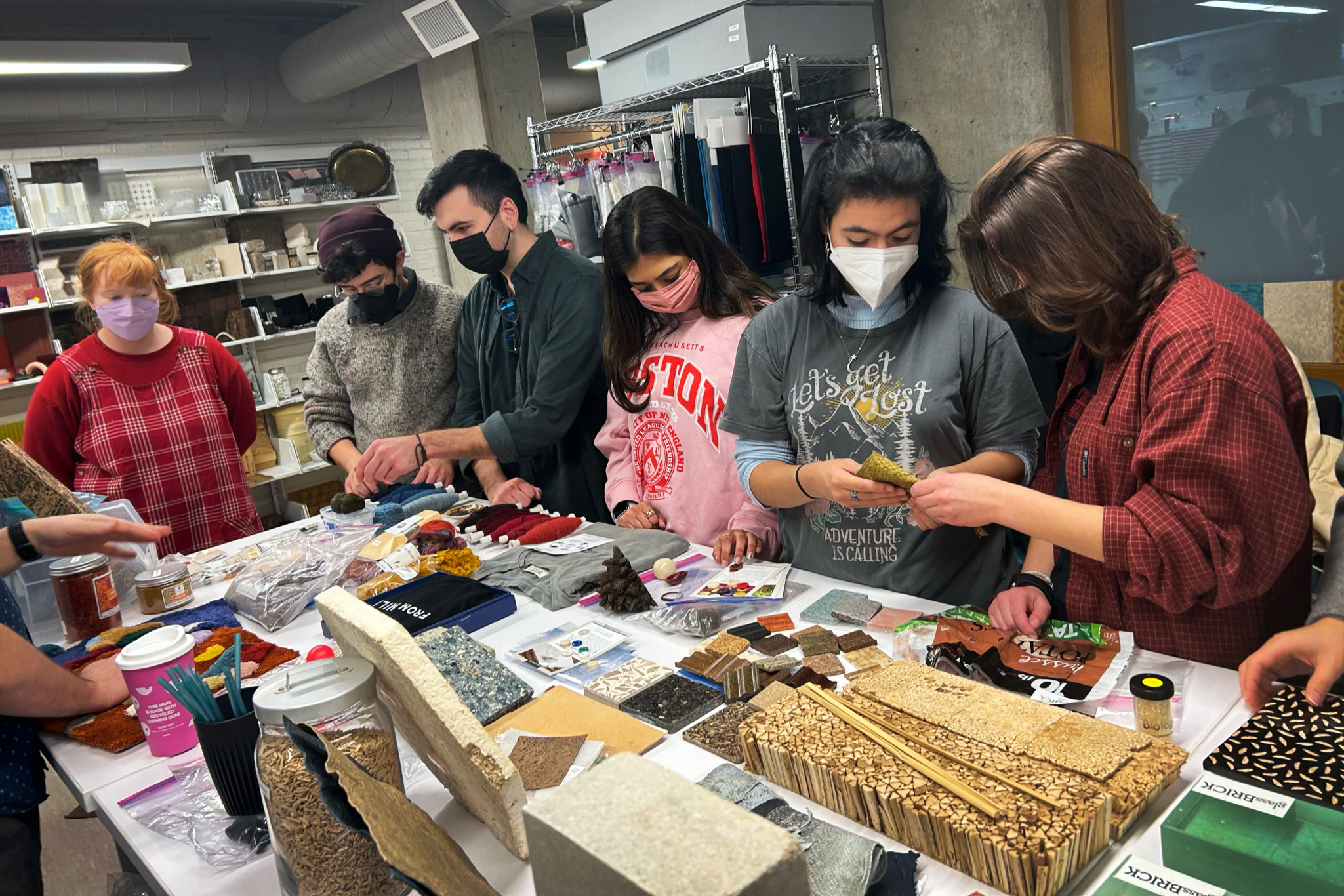In this image, six individuals, possibly students or a group involved in an art project, are gathered around a large table cluttered with various crafting materials. The room has an industrial feel, highlighted by visible ceiling ductwork and numerous shelves stocked with bins in the background. The table is laden with a diverse array of items, including cork and stone pieces, various fabrics and yarns in colors like red, burgundy, black, blue, and light gray, as well as jars filled with different materials, possibly rocks or pebbles, and even some glitter.

The group appears to be examining these materials closely, feeling them with their hands, which suggests a hands-on learning activity or a preparation for a crafting project. They are all wearing masks, indicating that the photo might have been taken during the COVID-19 pandemic. Among the group, a woman with red hair wearing a matching red top and dress is prominently visible on the left. Next to her is a man in a gray sweater and another man in a darker gray collared shirt. Additionally, there's a woman in a pink Boston sweatshirt, a woman in a gray "Let's Get Lost" t-shirt, and someone on the far right in a red checkered flannel shirt.

The overall atmosphere suggests an educational or creative session taking place in a space that could be a workshop or an arts and crafts retail store. The detailed assembly of materials and the participants' engagement reflect a thorough and interactive environment.